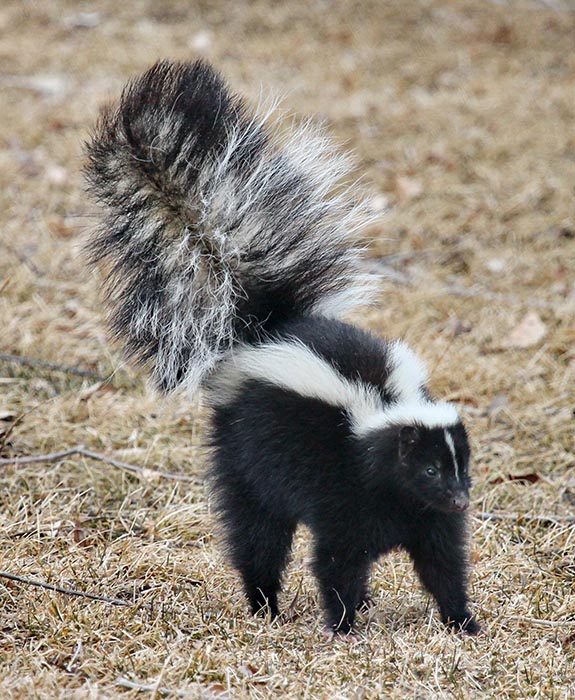The image captures a detailed close-up of a small, black-and-white skunk standing on a ground littered with dry, brown grass, twigs, and sticks. The skunk, facing forward, features a small head with a black nose and eyes. A prominent white stripe starts at the top of its head, runs down its face, and splits into two down its back. The skunk’s bushy tail, raised high in the air, showcases a mix of black and white fur, adding to the overall fuzzed-out appearance of its coat. The setting is devoid of any other animals, trees, or human elements, emphasizing the secluded, natural environment.